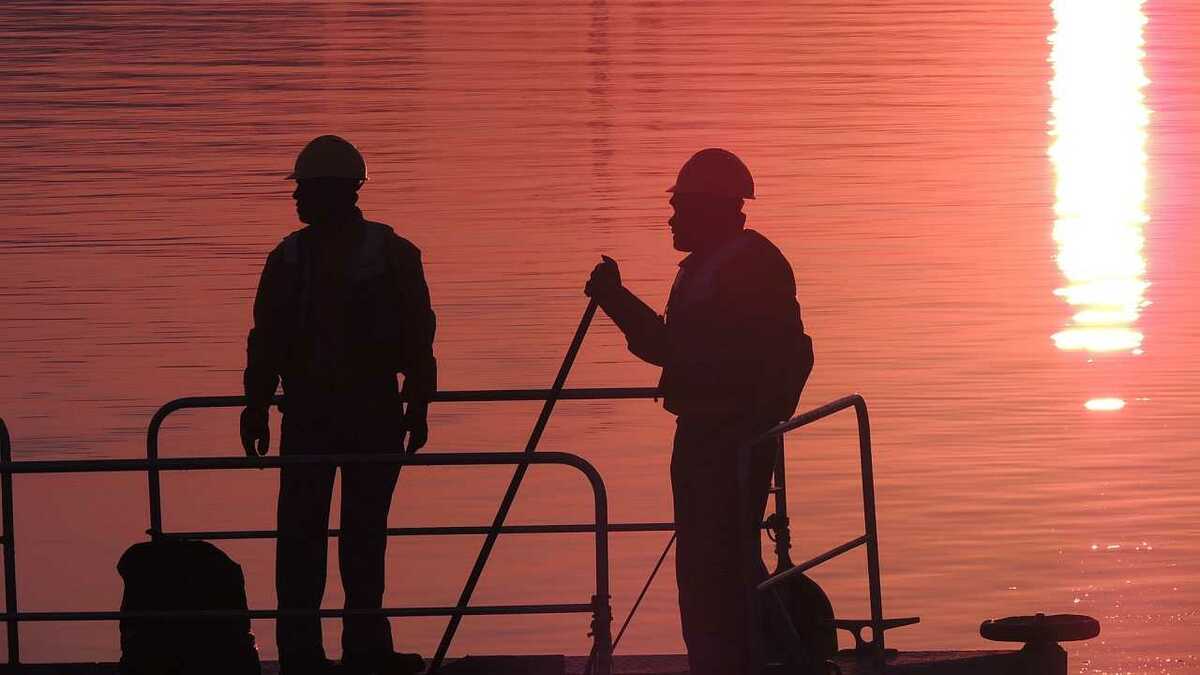In this image, two men are positioned on a platform that appears to be part of a boat, set against a serene body of water at sunset. The water, reflecting the sunset, casts a warm, reddish-orange hue over the scene, rendering the surroundings in an ethereal glow. Both men are workers, identifiable by their hard hats—one in yellow and the other in reddish-orange—and jackets adorned with company emblems. They stand within a bounded space featuring railings along the front, sides, and back. The man on the right grips a long pole that extends into the water, perhaps as a navigational tool, suggesting that the platform might indeed be a boat. Nearby, a filled trash bag rests beside the man on the left. The calm water is slightly rippled and mirrors the diminishing sunlight, adding to the tranquil yet industrious atmosphere.